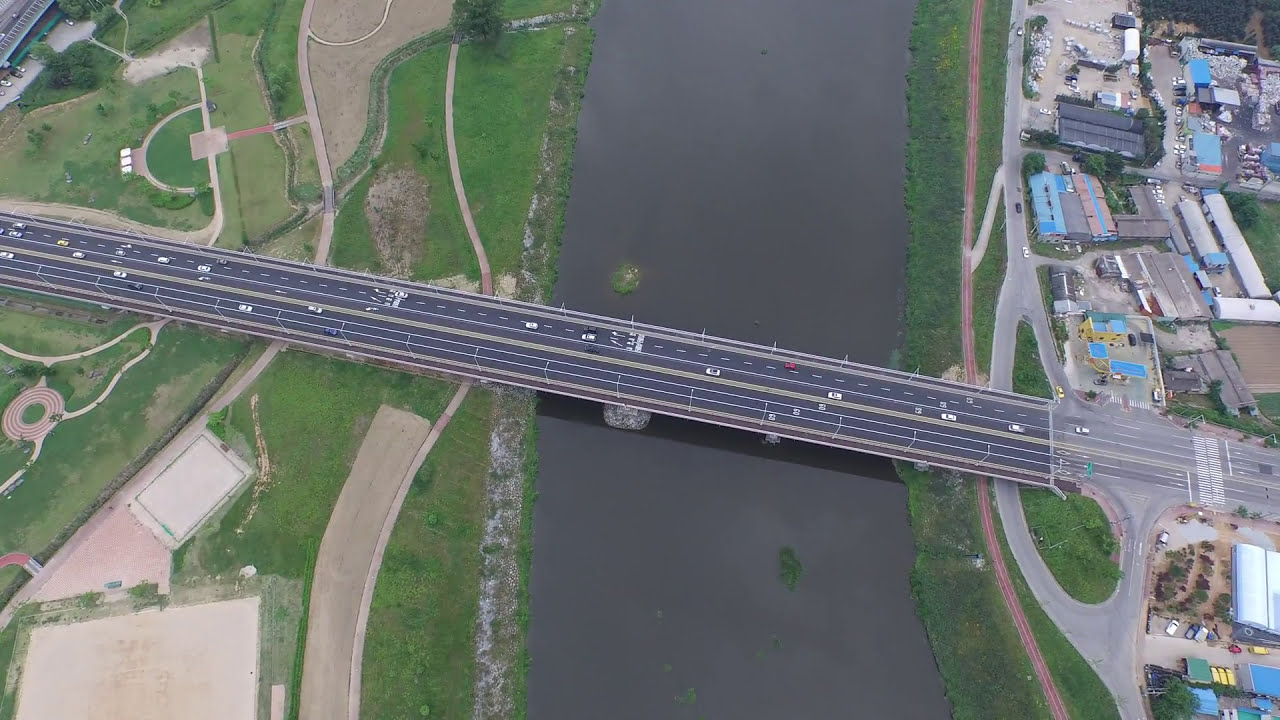This is an aerial photograph of a six-lane highway bridge spanning over a dark gray, possibly muddy river or canal. The bridge accommodates traffic in both directions and features distinct white lane markings. On the left side of the bridge, there is a verdant area marked by green grass, trails, dirt paths, and some circular roundabouts, giving the appearance of a park-like or possibly agricultural landscape. The right side presents a stark contrast with its industrial park comprising tightly packed, long pole buildings—like those used for storage or factories—distinguished by blue and green roofs. This area is bustling with activity, featuring parking lots, big yellow semis, white work trucks, piles of stone, and tarps, reinforcing the industrial ambiance. Roads run perpendicular to the bridge, connecting the on and off-ramps to the surrounding grid.